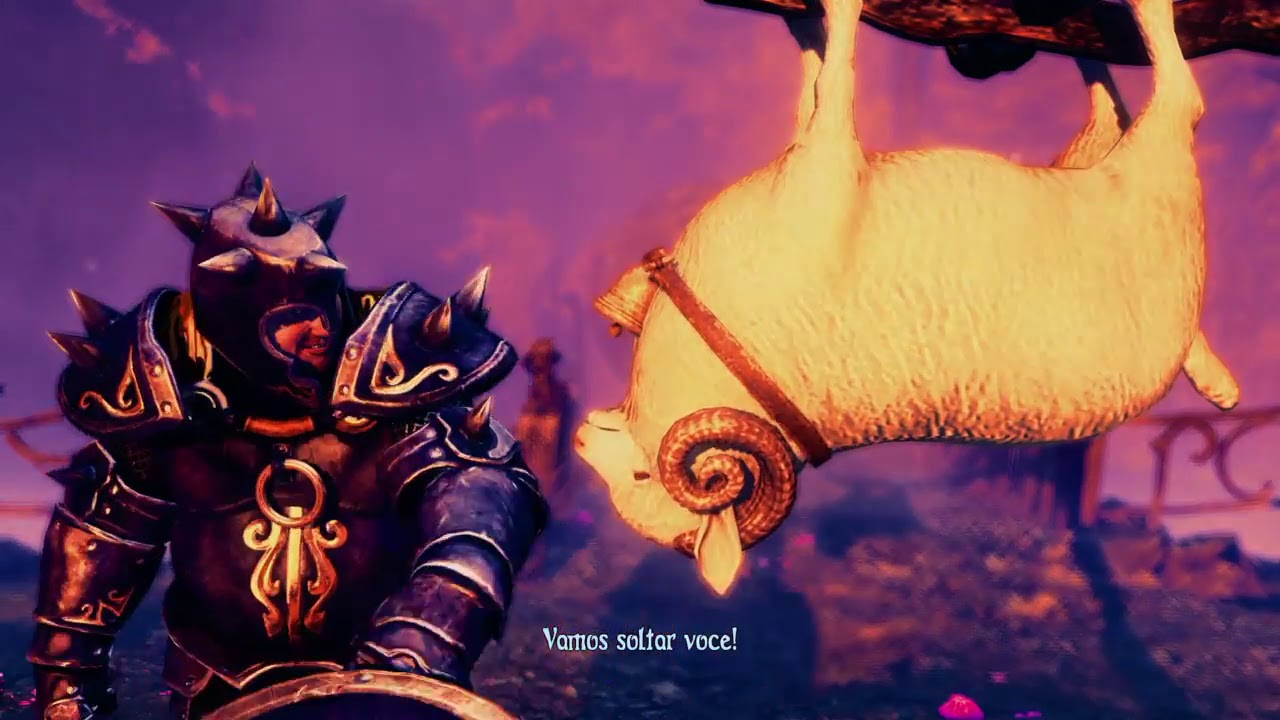The image appears to be an intricately detailed, digital or painted scene, inspired by old movies or graphic novels. On the left side of the landscape-format image, a knight dressed in elaborate, spiked armor stands from the waist up, gazing towards the right. His armor is adorned with menacing spikes on his helmet and shoulders, and he sports a round, gold-red design on his chest resembling a child's head and body. The knight holds a shield in his right hand while his left hand remains partially hidden. His battle-ready ensemble hints at a state of readiness for combat.

To the right side of the image, an upside-down ram, reminiscent of claymation with white fur and curved horns, hangs from a tree branch by all four limbs. The ram wears a brown belt with a bell around its neck. The background of the scene is a surreal blend of purple, light orange, and pink hues, creating a glowing, ethereal atmosphere. At the bottom center of the image, small white text reads "Vamos Soltar Voce," adding a cryptic element to the composition. The combination of these elements lends the image a fantastical and mysterious quality, leaving viewers intrigued.